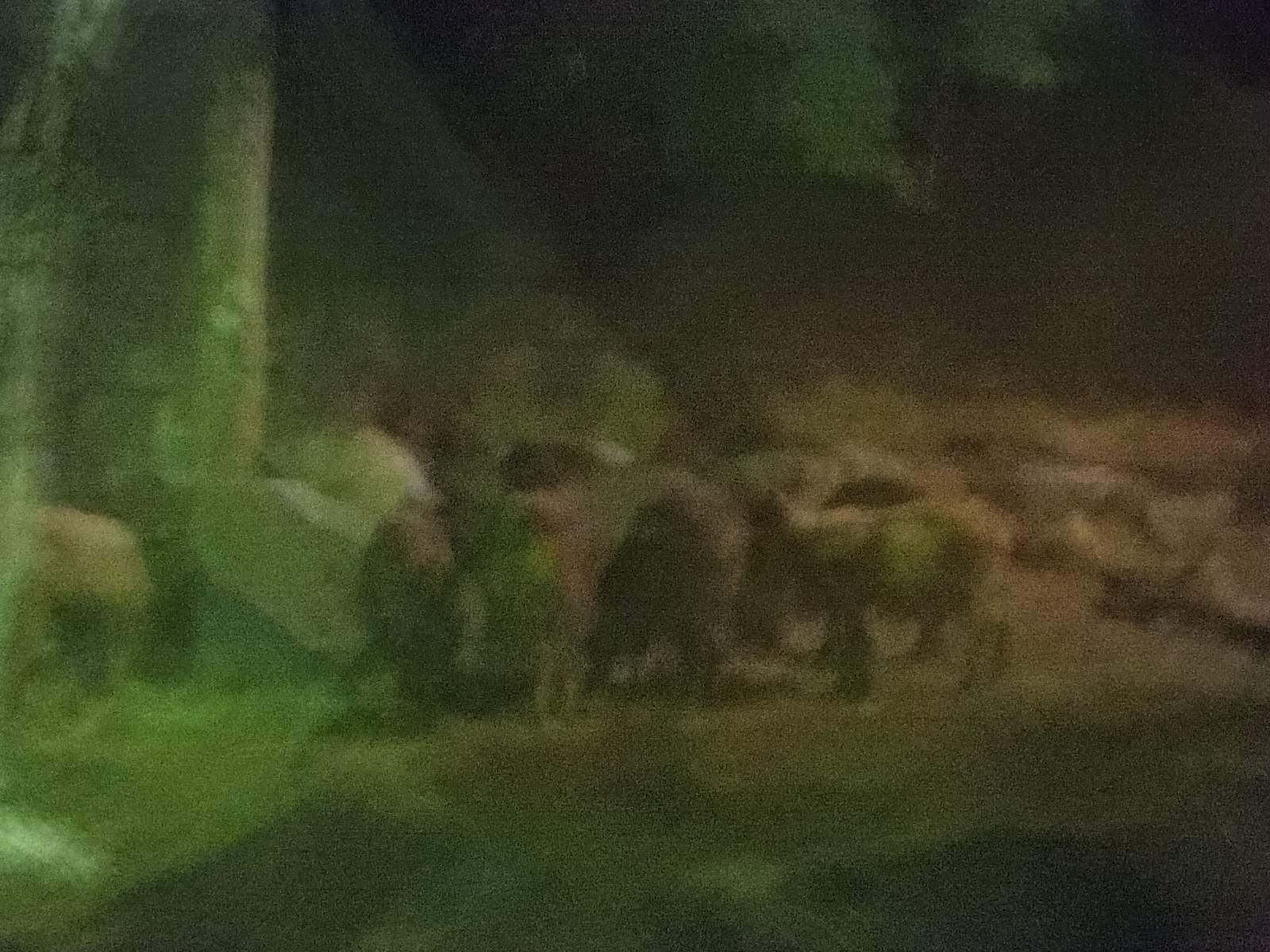This image, despite its grainy and unfocused quality, presents a scene reminiscent of early art from cave paintings or low-resolution video games. Central to the composition is a herd of animals, several of which resemble elephants, suggesting they could be mastodons or similar prehistoric creatures. Among them, a few animals carry the shapes of horses or early cattle, emphasizing the ambiguous nature of the depiction.

The setting appears to be inside a cavern, characterized by imposing rock pillars on either side, with rough boulders and stubble scattered in the background. The dark overhang and shadowy depths further enhance the cave-like environment, contributing to a sense of primordial mystery. A cliff occupies the foreground, adding a sense of depth and terrain variability to the scene.

Notably, a possible human figure stands in the center, clad in what seem to be furs or skins, suggesting early human interaction with these creatures. The overall color palette of the image is dominated by dark greens and blacks, reinforcing the vintage and ancient atmosphere of this evocative and enigmatic tableau.